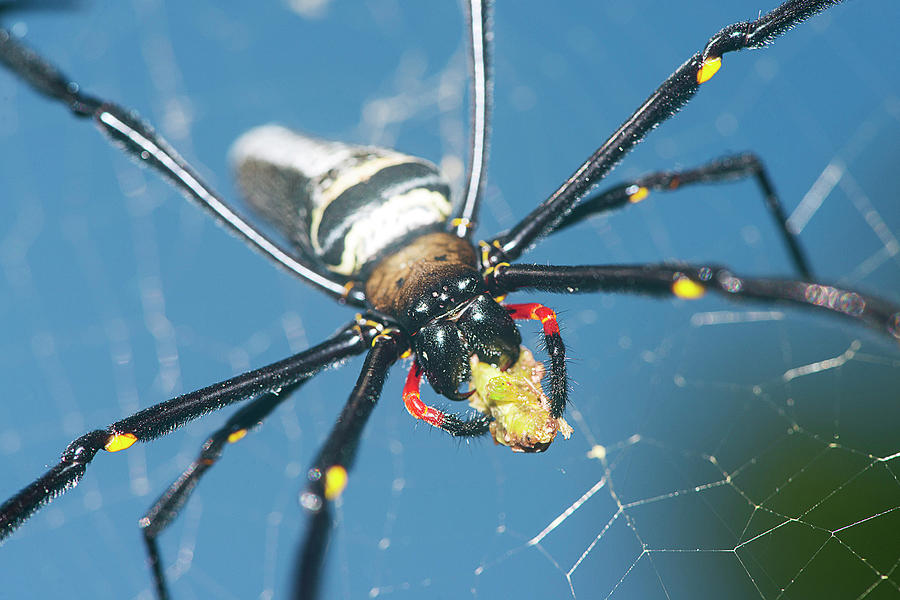This is a highly detailed, close-up photograph of a spider devouring its prey on its web. The spider, with eight legs, dominates the frame, its legs extending beyond the edges. The creature's body is intricately colored and textured. It has a brown thorax featuring two black spots, and its mouth parts, known as pedipalps or chelicerae, are black with red arm sections capped in fuzzy black tips. The legs are primarily black, adorned with yellow at the joints and knees, and are covered in noticeable hairs. The spider’s head has red and yellow marking near its face, and it seems to be facing slightly toward the camera. The abdomen, although out of focus, appears brown with potential yellow and black banding.

The web is subtly visible, catching light primarily in the center under and behind the spider, but it becomes blurry towards the edges. The prey it is consuming is light brown with tinges of green and darker brown segments. The image's background is overwhelmingly out of focus, hinting at a blue sky and some green foliage, which further emphasizes the spider in its intricate web. The extreme close-up magnifies the spider to a nearly grotesque level, showcasing every hairy detail and evoking a sense of both awe and unease as the spider feasts.